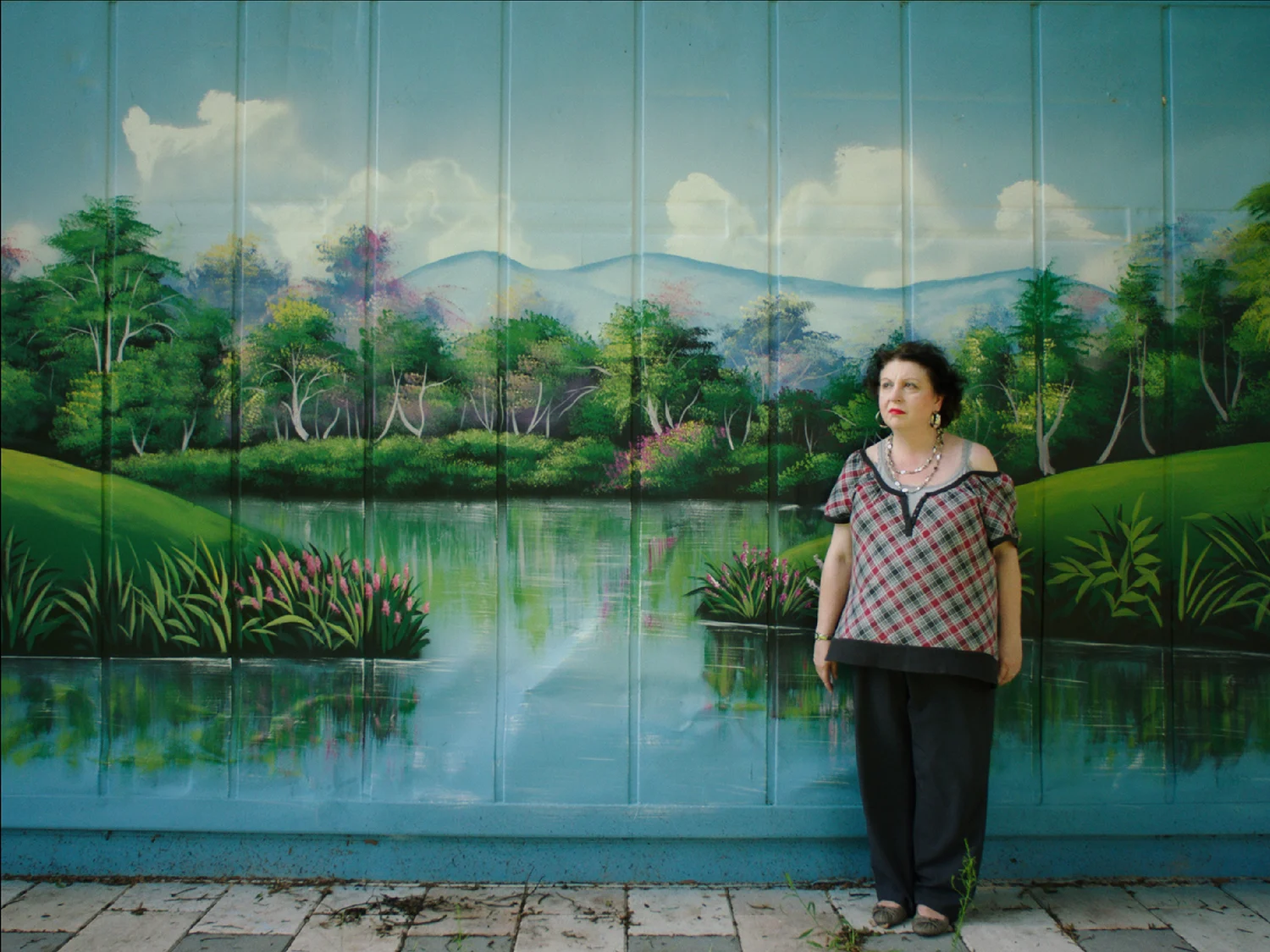In the image, a middle-aged woman stands against a wall adorned with an extensive and colorful mural. The mural depicts a tranquil lake surrounded by lush green grass, trees, and bushes, with splashes of vibrant pink flowers. The background features a distant mountain range under a bright blue sky filled with fluffy white clouds. The woman appears to be gazing off into the distance, as if uninterested or unprepared for the photograph.

She is wearing a top with a crisscross or checkered pattern in shades of red, black, and white, and black pants. Her shoes are flat, possibly silver in color, and she does not wear socks. Her attire is accessorized with multiple necklaces and prominent, large earrings. Her straight black hair frames her face, completing her casual yet distinctive look. She stands on a concrete pavement scattered with some dried branches, possibly from nearby plants, enhancing the earthy feel of the scenery.